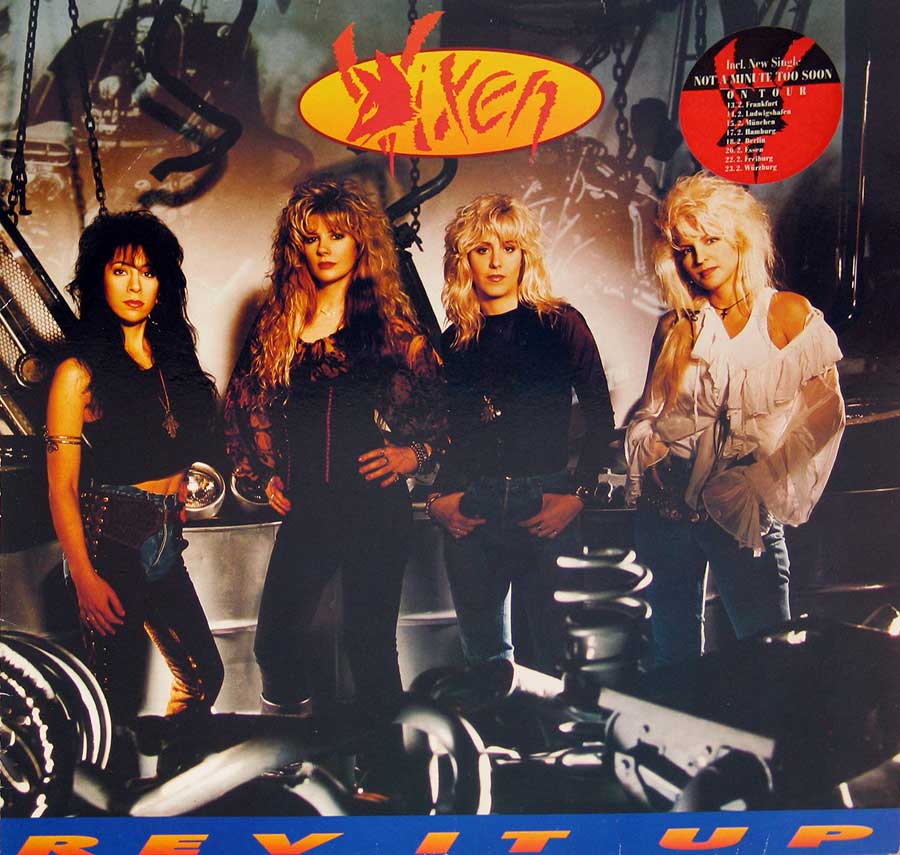The image depicts the cover of a CD or vinyl record by the all-woman band Vixen. The band's logo, featuring the word "Vixen" in a gritty, reddish-orange stylized font with a fox head over the 'V,' is prominently displayed at the top. The cover showcases the four band members standing side by side, embodying a quintessential 80s rock aesthetic. The first woman on the left has dark hair and is dressed in a black top with studded leather pants or chaps over blue jeans. The second woman is a darker blonde, sporting a crimson top and black pants. The third woman, also blonde, wears a purple shirt and blue jeans. The woman on the far right is a light blonde with teased hair, donning a white blouse and blue jeans. The background appears to be a mechanic's shop, filled with metal parts and motorcycles, enhancing the rugged and rebellious vibe. A distinctive blue strip at the bottom of the cover reads "Rev it up." In the top right corner, a black and red sticker provides additional information, including a note about their latest single and tour dates.